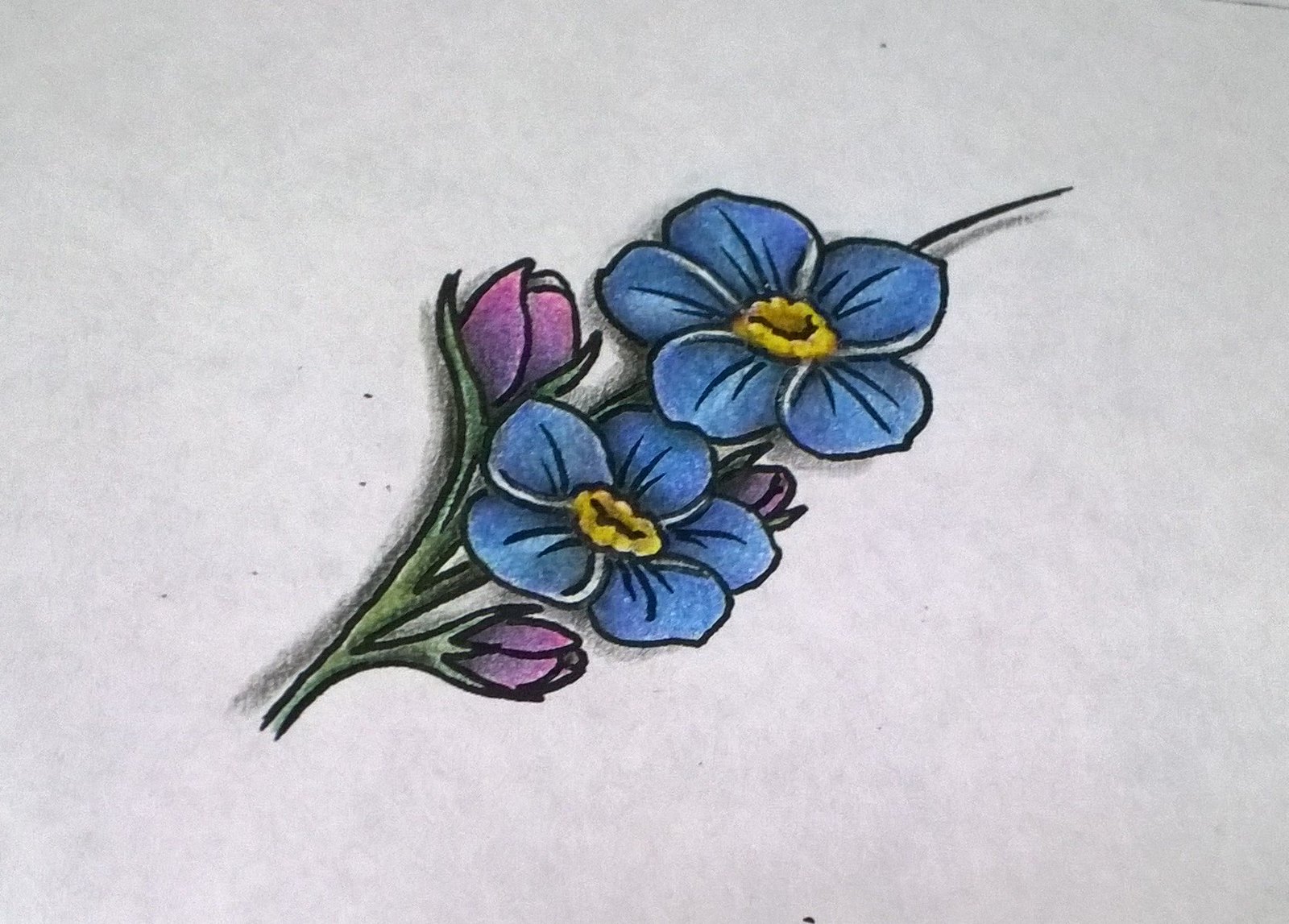The image features an intricately detailed drawing or painting with a tattoo-like aesthetic set against a white background. The artwork depicts a flower with meticulous attention to detail, suggesting the use of colored pencils, although it could also be paint. The composition starts with a green stem, leading upward to reveal several purple buds. Further along the stem, fully open blue and yellow flowers are rendered with exceptional shading that creates a realistic illusion of shadows cast on the surface. The vividness and precision of the colors highlight the artist's skill, making the floral depiction both vibrant and lifelike. The image is purely visual, with no accompanying text.